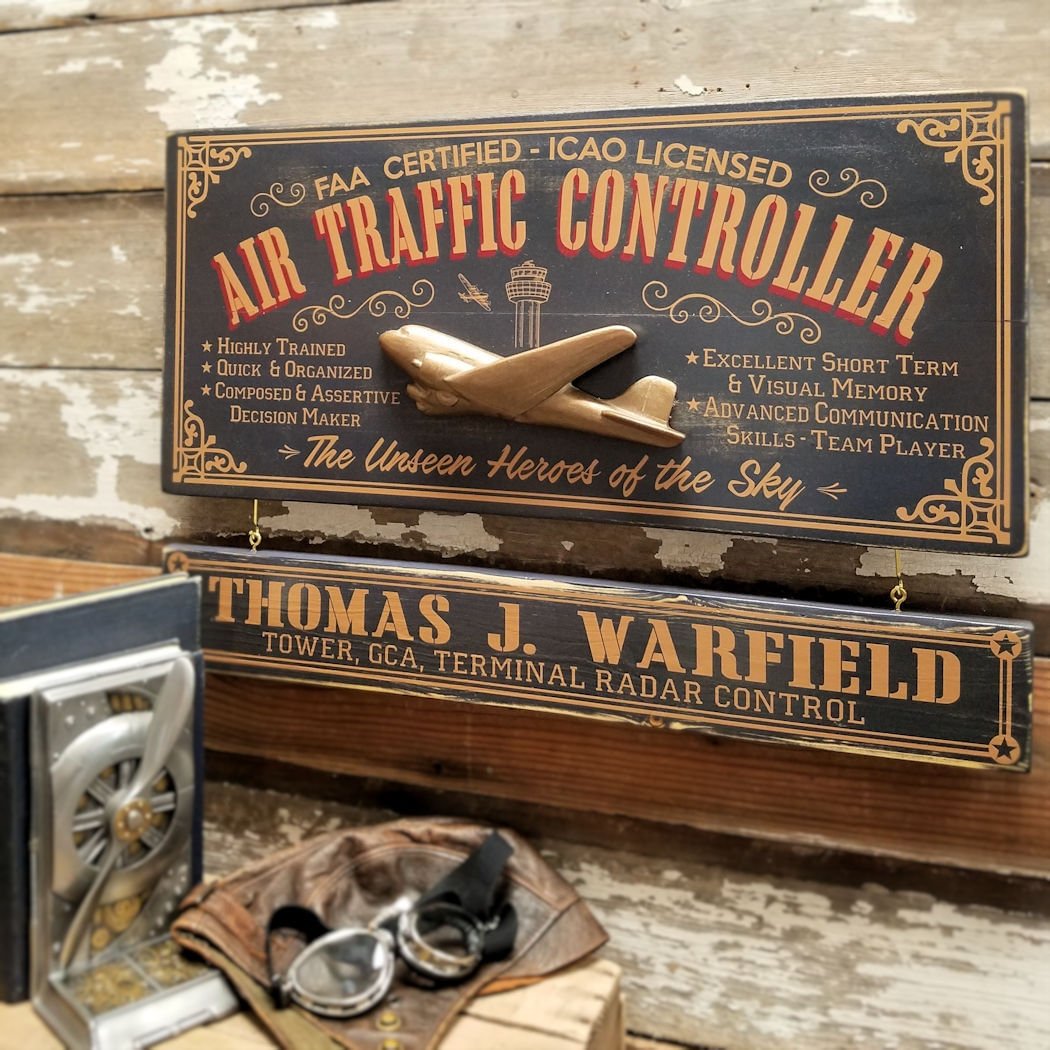The image is a color photograph in a square format that prominently features memorabilia dedicated to air traffic controllers, with a particular focus on Thomas J. Warfield. Centrally placed against a weathered wooden wall made of individual planks are two notable signs. The larger, topmost sign has a black background adorned with gold-colored filigrees at each corner and prominently displays in bold, dark cream-colored text with a red drop shadow reading "FAA Certified, ICAO Licensed Air Traffic Controller." Below this in smaller, cream-colored text are bullet points: on the left, "Highly Trained, Quick and Organized, Composed and Assertive Decision Maker," and on the right, "Excellent Short-Term and Visual Memory, Advanced Communication Skills, Team Player." At the center and near its bottom is a 3D sculptured model of an airplane in flight, nose pointed to the top left, with an illustration of a control tower behind it. In a stylish script below the airplane, the text reads, "The Unseen Heroes of the Sky." Hanging below this larger sign, on chains, is a smaller sign that reads, "Thomas J. Warfield, Tower GCA Terminal Radar Control." 

In the foreground, slightly out of focus, lie several pieces of aviation paraphernalia on the bottom left, including a pair of aviator glasses and a brown leather cap. There appears to be some kind of metallic device, possibly an old aviation instrument with a propeller. The photograph, stylistically categorized under Photographic Representationalism Realism, evokes a sense of historical reverence, suggesting either a memorial plaque or a recreation of an air traffic controller's workspace from approximately 80 to 90 years ago.